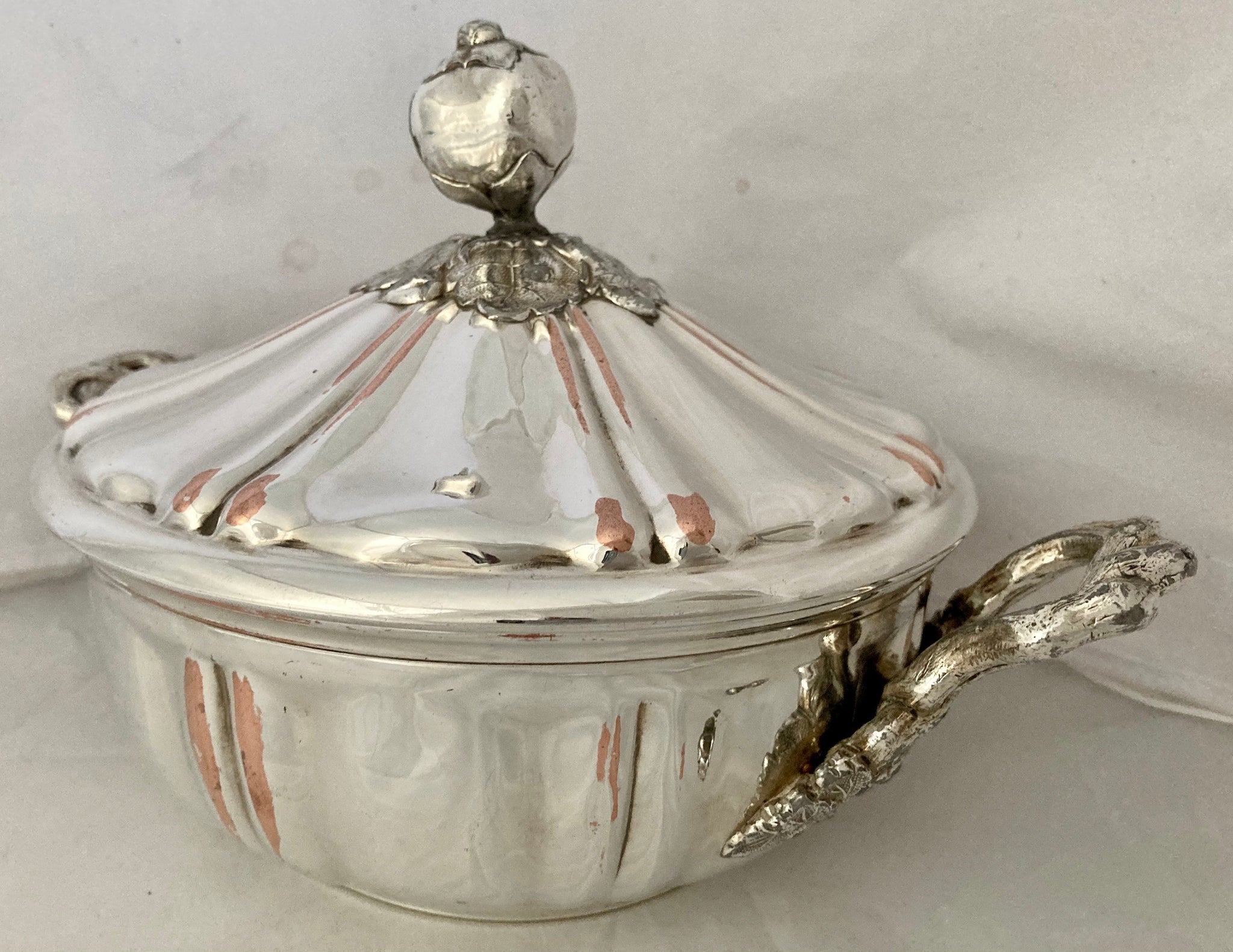The image features a shiny, ornate silver serving dish positioned centrally on a white, slightly rippled cloth backdrop. The elegant round dish has a dome-shaped, pie-piece designed lid that arches upward. At the top of the lid, there is an eye-catching, cherry tomato-shaped knob for lifting. Matching silver handles are attached to either side of the dish, which shares the same darker silver hue as the top knob. The backdrop gives a grayish appearance with slight wrinkling, providing a neutral contrast to the dish's brilliance. The cohesive silver aesthetic, from the decorative knob to the handles, unifies the image and showcases the refined beauty of the serving vessel.